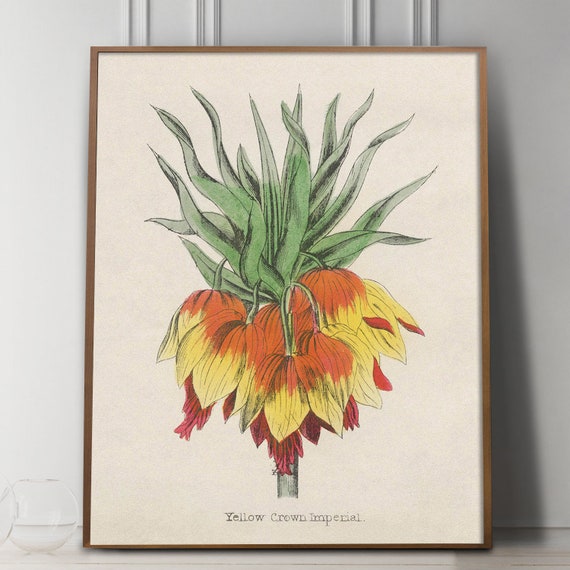The image features a detailed drawing of a plant known as the "Yellow Crown Imperial." The drawing, which appears to be created with pencil and possibly colored with watercolor, is set within a thin, brown wooden frame. The plant has numerous vertical, blade-shaped leaves transitioning from vibrant green to a gray-green hue. Hanging upside down from the stems are feathery flowers that display a gradient from orange at the base, through yellow in the middle, to red at the top. The drawing is propped against a very light gray wall adorned with vertical molding seams. The lower left corner of the image reveals two half-filled water glasses resting on a light hardwood floor. The wall behind the picture gradiates from gray to very light gray, with some molding visible behind the framed drawing. At the bottom of the drawing, the text "Yellow Crown Imperial" identifies the plant.